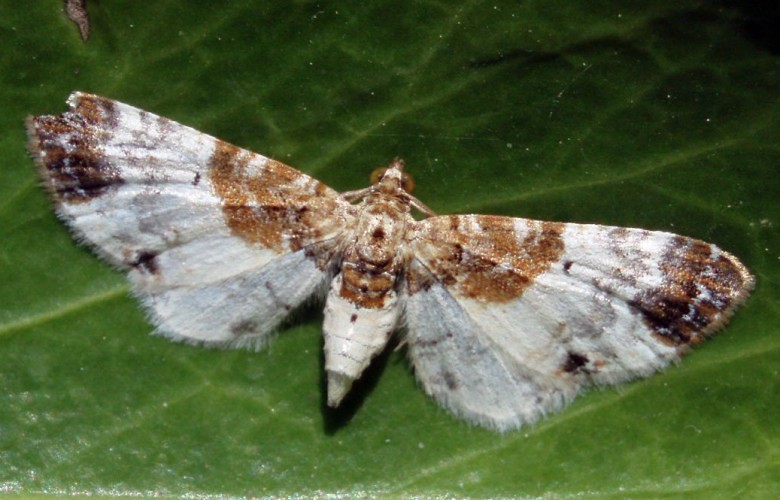This detailed, color photograph captures a moth resting on a leaf, with the leaf filling the entire background of the image. The photograph, in a landscape orientation, shows the leaf's asymmetrical dark and light green hues, transitioning from dark green in the upper right-hand corner to a lighter shade in the bottom left-hand corner, where reflections of light can also be seen. The leaf's veined texture provides a naturalistic backdrop that emphasizes the moth's delicate features.

At the center of the image, the gray moth is showcased with its wings fully outstretched, running diagonally from the top left to the bottom right. The moth's body exhibits a tapered, symmetrical design, adorned with shades of brown and white. The patterns on its wings, also symmetrical, present various shades of brown converging toward the body's base. The wings' edges feature fine, hair-like fibers, giving a fringed appearance, with dark brown tips. Two small, round brown eyes and short antennae add to the intricate detailing of the moth. The style of the image is a clear example of photographic representational realism, capturing the intricate beauty of the moth and its natural habitat.